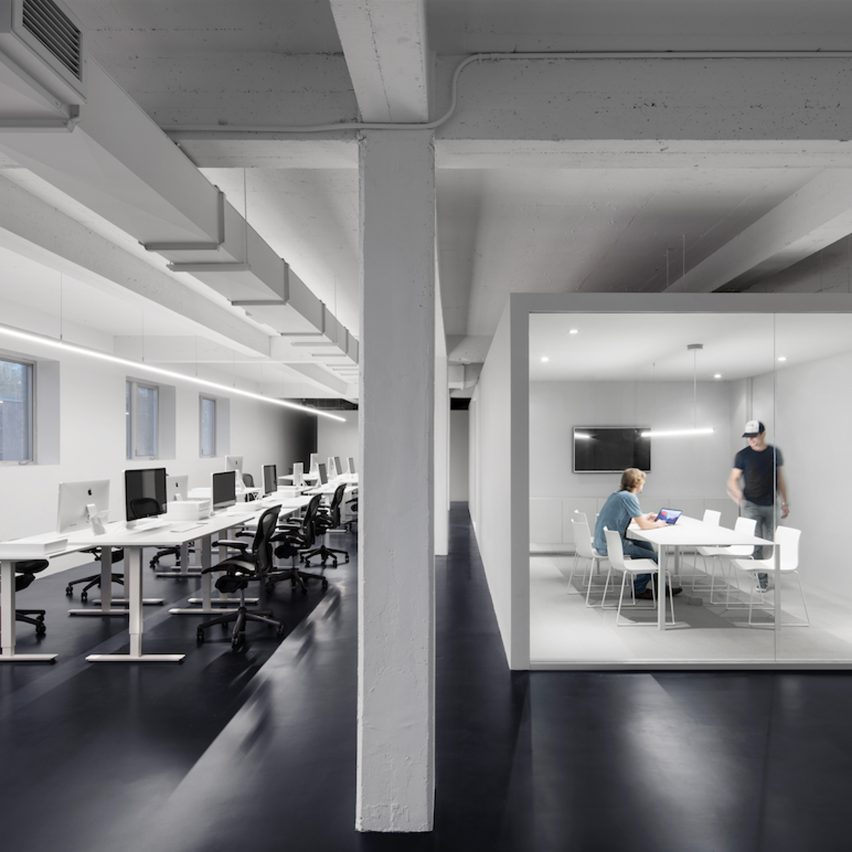This image depicts a very modern office space, characterized by its sleek, contemporary design and open warehouse-like setting. On the left side of the room, there is a long white table lined with workstations fitted with black monitor screens displaying the Apple logo, some of which are silver in color. These workstations vary in height, supported by T-shaped legs that extend to the floor. The chairs in front of these desks are thin, black computer chairs that complement the white desks.

The office features a glossy black floor, adding to the modern aesthetic, and walls painted white, with three windows that are slightly raised and closed. A divider or pillar splits the room, separating the workspace area on the left from a meeting room on the right.

The meeting room is enclosed with windowed glass and contains a conference table surrounded by six white chairs that match the desks outside. A flat-screen TV is mounted inside the meeting room.

In the center of the scene, near the divider, are two young men. One is seated at a workstation, dressed in a green t-shirt, with brownish hair, focused on his laptop. The other man, wearing jeans, a t-shirt, and a baseball hat, is standing nearby, engaging in conversation. The overall color scheme of the office is dominated by white, gray, and black tones, emphasizing its modern and corporate Apple-like atmosphere.